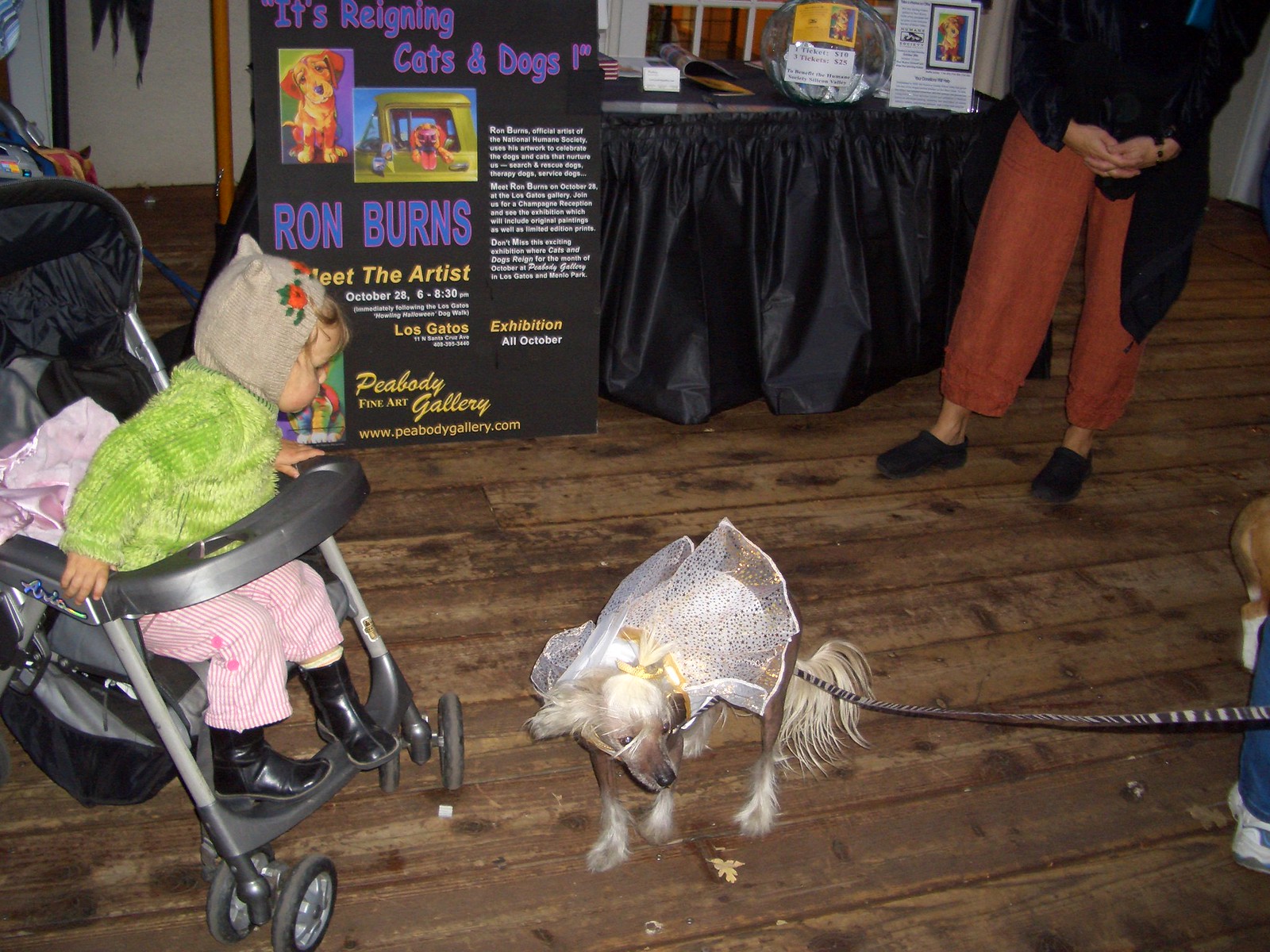In the foreground, a small white dog, possibly wearing a wedding veil or angel wings, stands on a horizontally-laid hardwood floor. The dog is on a leash held by someone off-camera to the right. Central to the image, a toddler girl of Caucasian descent leans over the front of a black and silver stroller, eyeing the dog with curiosity. The girl is dressed in pink and white striped pants, a green coat with a gray hood adorned with cat ears, and black boots.

In the background, a table with a black skirt displays a fishbowl and a plaque. To the left of the table, a black poster with purple and yellow text announces, "It's Raining Cats and Dogs! Meet the Artist, Ron Burns." The promotional details include an exhibition date of October 28th from 6 to 8:30 p.m. at the Peabody Gallery in Los Gatos. Partially visible behind the table is a woman dressed in orange pants and a black long-sleeved shirt, with her arms folded. The scene suggests an indoor event or exhibition, captured with a focus on the interactions between the child and the dog.